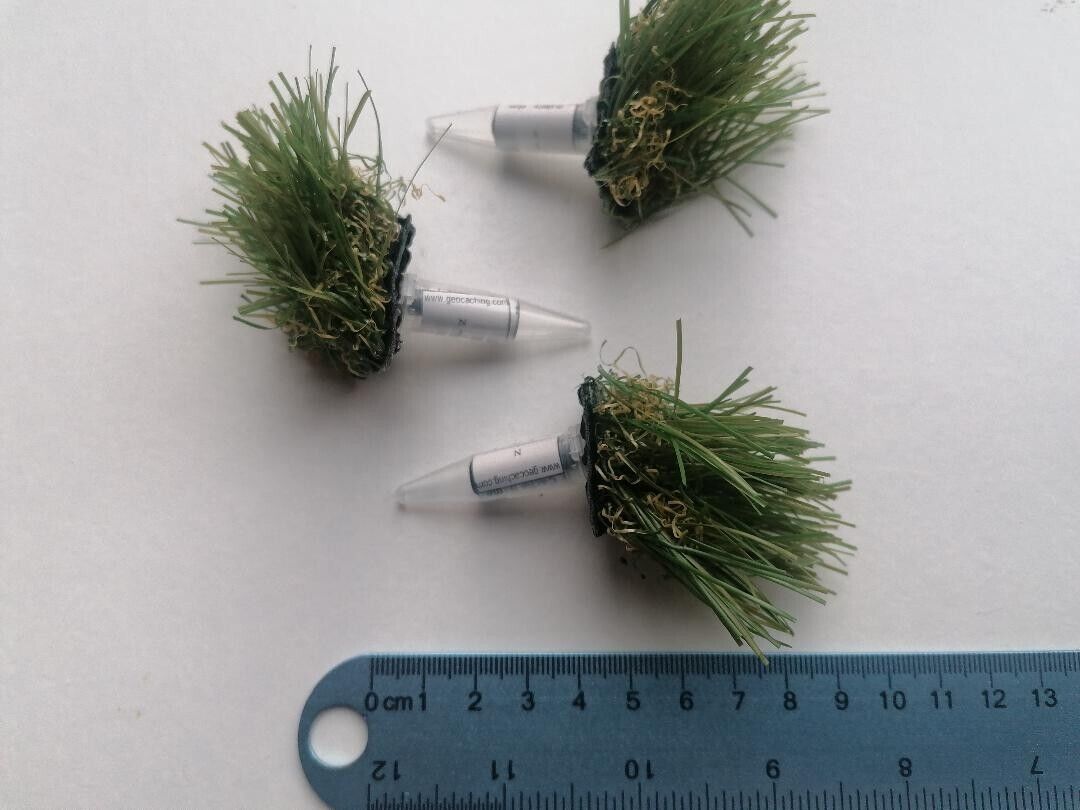The image displays three transparent plastic vials, each topped with artificial grass tufts, arranged against a white background. The vials have small labels wrapped around them, one of which appears to bear the partially readable URL "www.geocaching.com". Each vial is affixed with grass that includes green blades and some brown, curly strands at the bottom. The vials are positioned alternately, with the first vial pointing to the left, the second to the right, and the third back to the left. Beneath these vials lies a blue ruler, featuring both metric (centimeters) and imperial (inches) measurements. The ruler extends almost entirely across the width of the image and features a semicircular hole at one end, presumably for hanging. The scene is meticulously arranged on a white surface, emphasizing the clarity and details of each object.